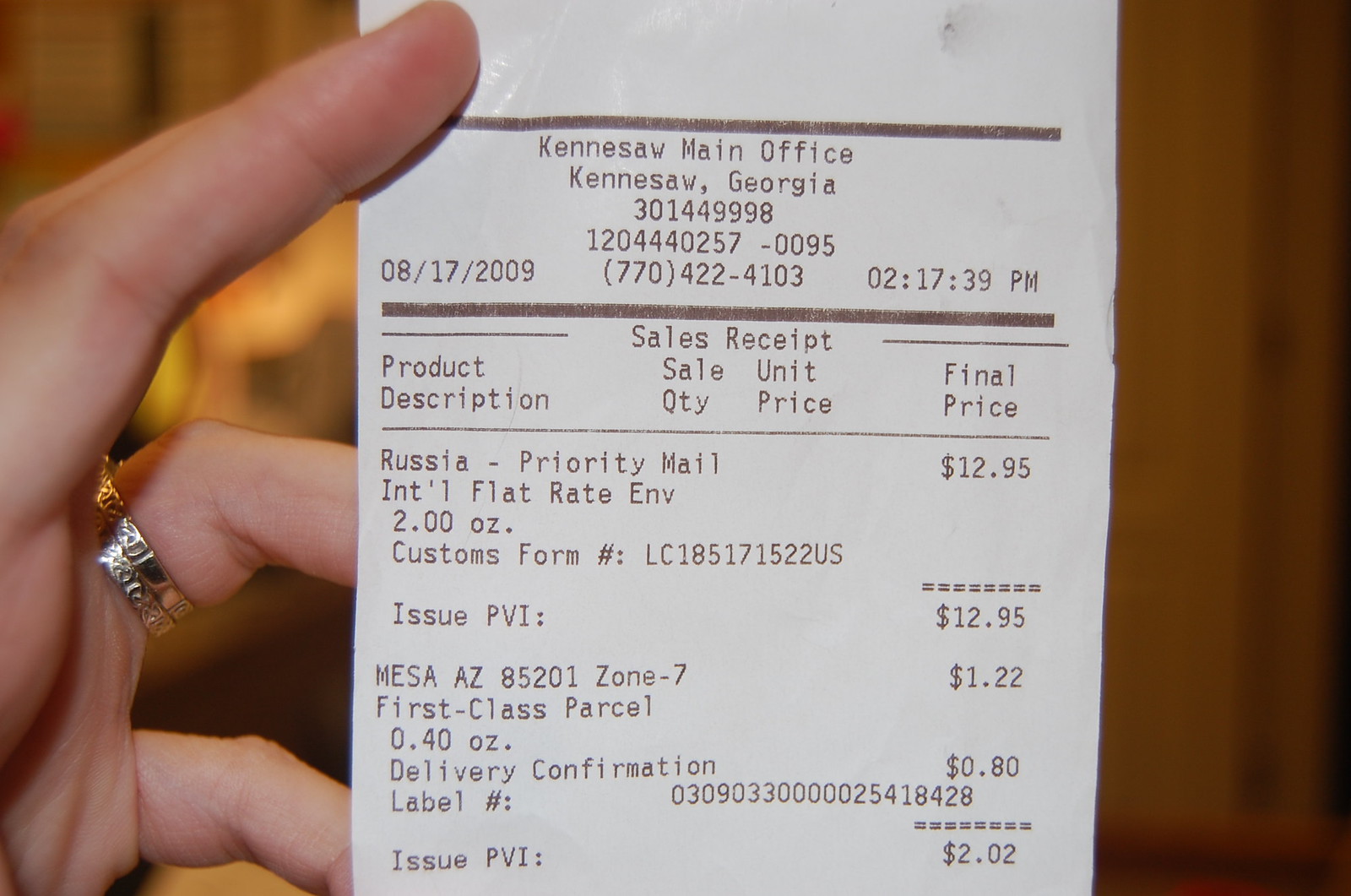The image depicts a digital photograph of a Caucasian person's left hand holding up a white sales receipt, prominently positioned in the center. The hand, adorned with a distinctive silver two-banded ring on the middle finger, contrasts against a blurred, tan background that resembles wood grain, indicating the photo was taken indoors. The receipt, printed with black text, is from the Kennesaw Main Office in Kennesaw, Georgia, with a detailed date of August 17, 2009, and a timestamp of 2:17:39 p.m. The main body of the receipt lists various shipping charges: $12.95 for Priority Mail International to Russia, $1.22 for a First Class package to Mesa, Arizona, Zone 7, 80 cents for delivery confirmation, and $2.02 for an issue PVI. The receipt includes customary columns such as Product Description, Sale, Quantity, Unit Price, and Final Price, underscoring the detailed transactional information.